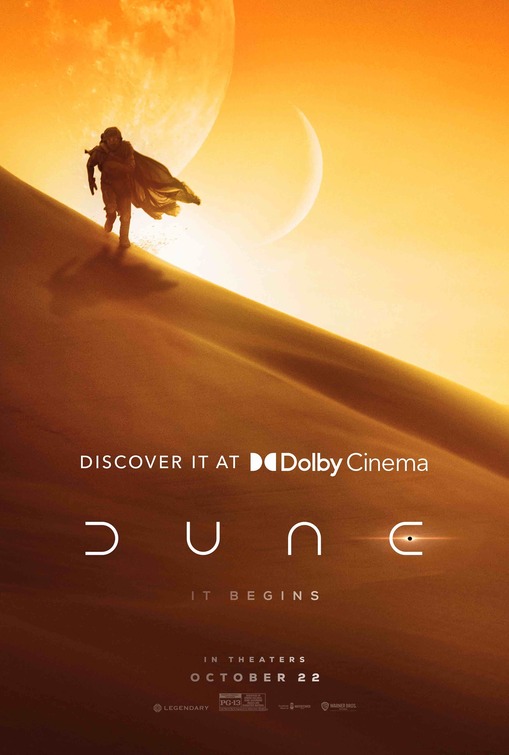This is a detailed movie poster for the sci-fi thriller, "Dune," prominently featuring a sweeping sand dune. Rising from the right side up to the left, the angle of the dune creates a dramatic backdrop against a vibrant, bright yellow sky. In the center, the poster showcases the text "Discover It at Dolby Cinema," followed by the movie title "Dune" in stylistic white print. Beneath the title, the tagline "It Begins" is stated, and further below, it specifies, "In Theatres October 22nd," along with a PG-13 rating and logos from Legendary and other studios.

In the image, a solitary figure clad in a flowing cape is captured walking along the sand dune, moving towards the viewer. The character is adorned with a head covering and sunglasses, signifying the harsh desert environment. Behind him, the sky hosts two celestial bodies—a dominant bright sun and a secondary, more distant planet or sun, adding an otherworldly element to the scene. The overall composition emphasizes the vast desert landscape and the impending epic narrative of the film.